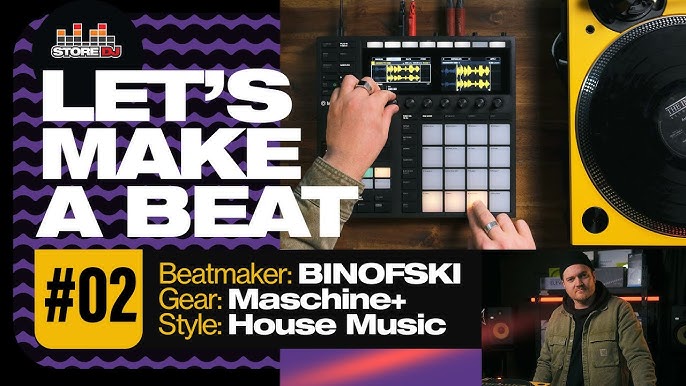In this digitally created collage, we have a landscape-oriented rectangular image brimming with various objects and images. Dominating the top left corner is a prominent sign that reads "Store DJ" above the bold white block letters "Let's Make a Beat." Just below this, in black letters on a yellow square background, is the hashtag "#02". Below this, in a black rectangular section stretching from the left to the middle bottom, the text reads "Beatmaker: Beinofsky," "Gear: Machine Plus," and "Style: House Music."

At the center top of the picture, a person’s hands manipulate the knobs of an advanced digital beat-making device, which has three buttons lit up brightly. To the right, a yellow rectangular section features a set of black circular devices, likely part of the musical gear. In the bottom right corner, there’s an image of a man gazing at the viewer, clad in a thick brown jacket over a black sweater, topped with a black knit cap. The array of colors in the image includes purple, white, black, yellow, army green, pink, and violet, contributing to the vibrant, visually stimulating advertisement.